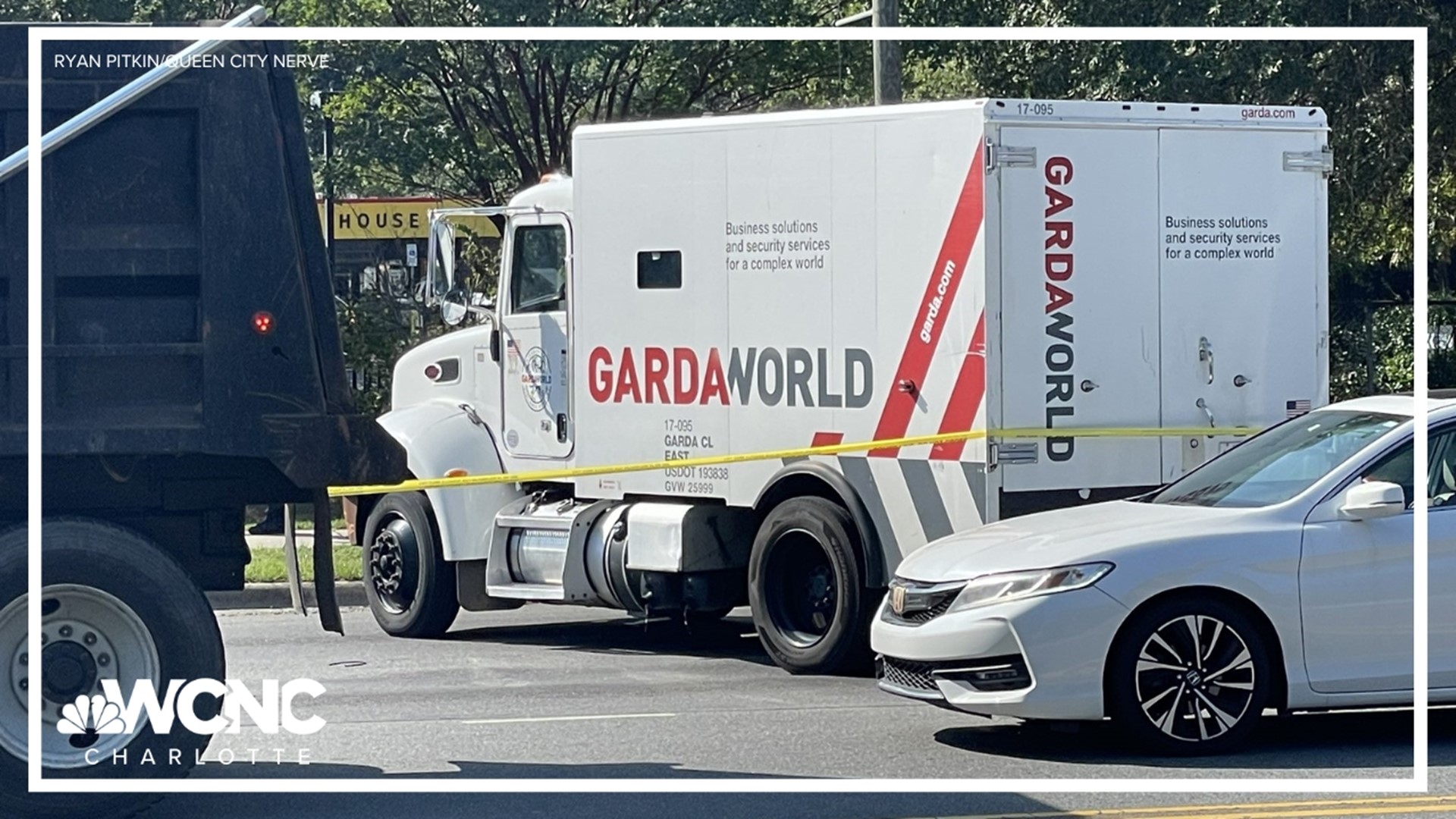The image is an outdoor photograph with a white border labeled "Ryan Pen Queen City Nerve." In the bottom left-hand corner, the caption "WCNC Charlotte" along with a peacock image suggests this is from a news company. Dominating the scene is a white Garda World armored truck, positioned at an angle on a roadway and showing a back three-quarter view. The truck displays the text "GARDA" in red and "World" in dark gray on its side, with two diagonal red bands. Additional text on the truck reads "Business Solutions and Security Services for a Complex World." The back of the truck also features "GARDA World" along with the same business slogan. In the foreground, partially obscuring the truck, is a white Honda car. To the left, the rear end of a black dump truck is visible. In the distance, a Waffle House sign is discernible. The area around the Garda World truck is cordoned off with yellow tape, suggesting a possible crime scene.